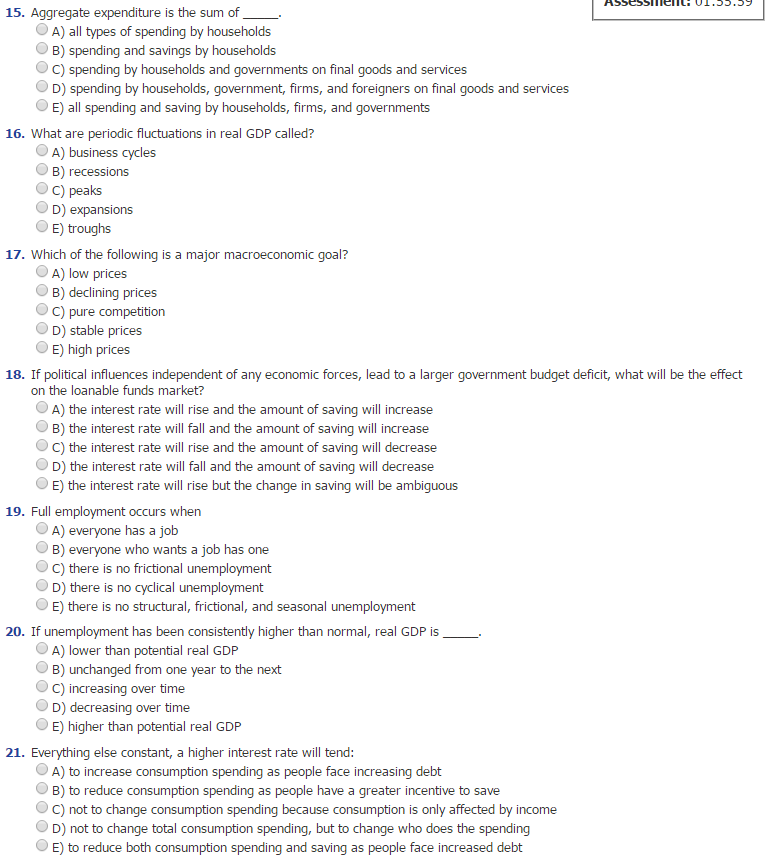The image is a screenshot of a multiple-choice assessment, likely a timed test, given the timer in the top right-hand corner that reads "Assessment: 155:59." The image displays questions numbered 15 through 21.

Question 15 asks, "Aggregate expenditure is the sum of":
- A) All types of spending by households
- B) Spending and savings by households
- C) Spending by households and governments on final goods and services
- D) Spending by households, government, firms, and foreigners on final goods and services
- E) All spending and saving by households, firms, and governments

Question 16 queries, "What are periodic fluctuations in real GDP called?":
- A) Business cycles
- B) Recession
- C) Peaks
- D) Expansions
- E) Troughs

Question 17 asks, "Which of the following is a major macroeconomic goal?":
- A) Low prices
- B) Declining prices
- C) Pure competition
- D) Stable prices
- E) High prices

Question 18 poses, "If political influences independent of any economic forces lead to a larger government budget deficit, what will be the effect on the loanable funds market?":
- A) The interest rate will rise and the amount of saving will increase
- B) The interest rate will fall and the amount of saving will increase
- C) The interest rate will rise and the amount of saving will decrease
- D) The interest rate will fall and the amount of saving will decrease
- E) The interest rate will rise but the change in saving will be ambiguous

Question 19 inquires, "Full employment occurs when":
- A) Everyone has a job
- B) Everyone who wants a job has one
- C) There is no frictional unemployment
- D) There is no cyclical unemployment
- E) There is no structural, frictional, and seasonal unemployment

Question 20 asks, "If unemployment has been consistently higher than normal, real GDP is":
- A) Lower than potential real GDP
- B) Unchanged from one year to the next
- C) Increasing over time
- D) Decreasing over time
- E) Higher than potential real GDP

Question 21 posits, "Everything else constant, higher interest rates will tend":
- A) To increase consumption spending as people face increasing debt
- B) To reduce consumption spending as people have a greater incentive to save
- C) Not to change consumption spending because consumption is only affected by income
- D) Not to change total consumption spending but to change who does the spending
- E) To reduce both consumption spending and saving as people face increased debt